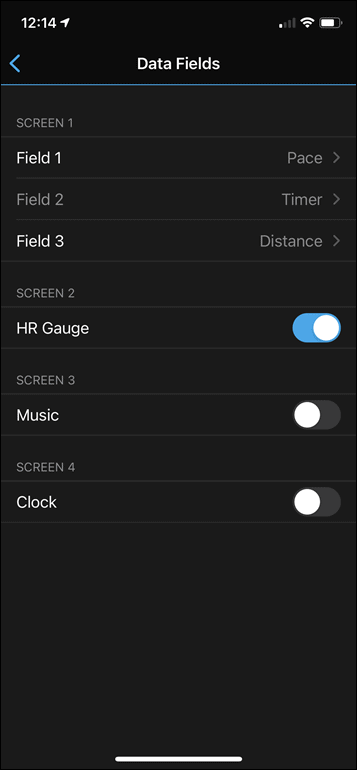Here is a cleaned-up and detailed caption for the given image:

---

This image, captured on an iPhone, shows a digital interface with various metrics and settings. In the top left-hand corner, the time is displayed as 12:14. On the upper right-hand corner, the signal strength bar indicates minimal connectivity with only one bar shown. The Wi-Fi icon displays full signal strength, and the battery indicator appears almost fully charged at around 90%. The background of the image is black.

At the center of the screen, there is a title that reads "Data Fields and Weight," separated by a blue arrow pointing to the left and a blue dividing line beneath the title. Below this header, the interface is divided into several sections labeled as "Screen 1," "Screen 2," "Screen 3," and "Screen 4."

Under "Screen 1," there are three columns titled "Field 1," "Field 2," and "Field 3." Each field has associated metrics:
- Field 1: Pace
- Field 2: Timer
- Field 3: Distance

Each metric (Pace, Timer, Distance) has an arrow pointing to the right, indicating further options or settings.

"Screen 2" displays "HR Gauge," which is toggled on. The toggle switch has a white circle positioned to the right and the entire toggle is highlighted in blue. 

"Screen 3" shows "Music," which is toggled off. Here, the white circle is positioned to the left, and the toggle switch appears in a gray-black color. 

"Screen 4" is labeled "Clock," also toggled off, with the same gray-black toggle and the white circle to the left. 

This comprehensive display offers a clear overview of various data fields and settings, providing detailed information on connectivity, battery life, and different configurable screens.

---

This caption offers a clear and structured description of the image, making it easy for readers to understand the various elements and settings shown.